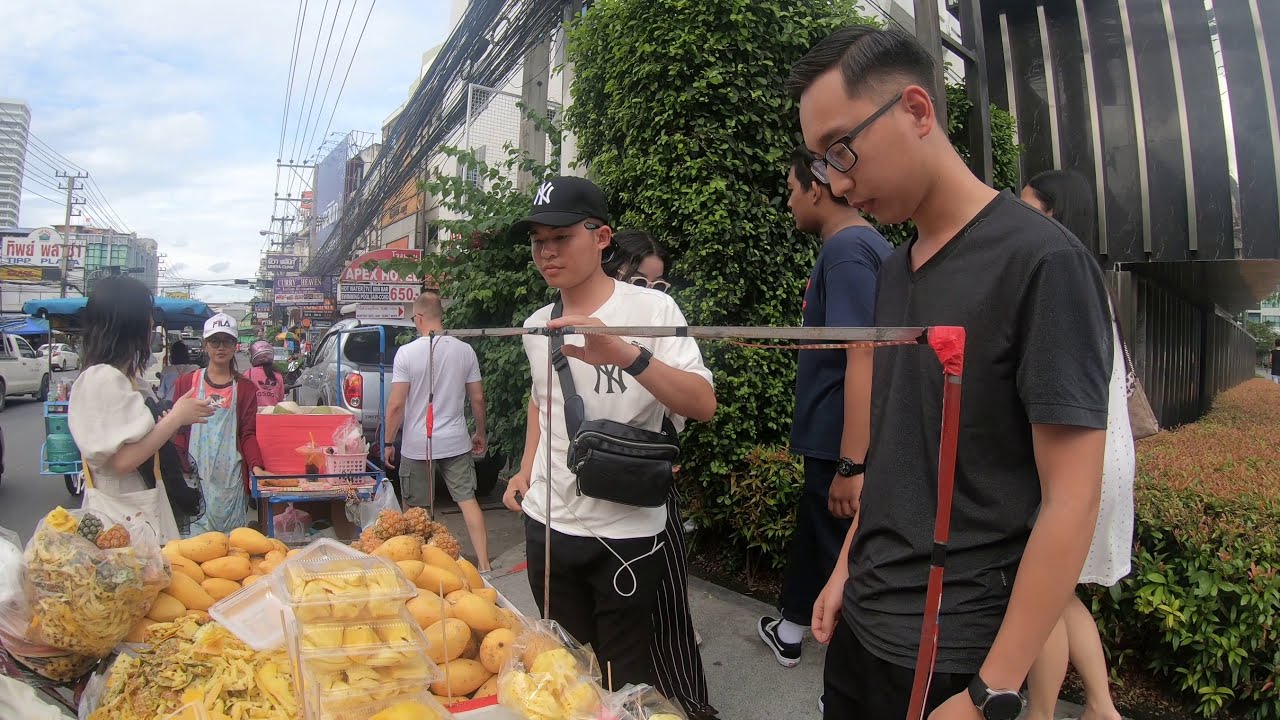In a bustling Asian city, under a bright blue sky filled with white clouds, a lively street market scene unfolds. The image captures a crowd of mostly Asian individuals gathered in front of a vibrant food stand, which is selling an assortment of fresh produce, potatoes, vegetables, and some bakery goods. The stand is managed by a woman wearing a blue apron, engaging with the customers in front of her. Among the crowd, a man in a gray shirt and glasses stands out on the right, while another man to his left sports a white t-shirt, black ball cap, and a shoulder bag paired with black pants. 

The backdrop consists of a mixture of buildings adorned with various signs, indicating nearby shops and stores. On the left, a woman in white, carrying a white purse, converses with another woman dressed in a ball cap and apron beside a table that holds a pinkish cooler. The roadway is a blend of foot traffic and car traffic typical of busy Asian urban centers, with parked cars visible in the background. Overhead, numerous wires stretch across the scene, contributing to the urban ambiance. The market tables overflow with stacked yellow vegetables, likely potatoes. In the midst of it all, a young man donning a New York Yankees baseball cap and a t-shirt stands, epitomizing the fusion of traditional and Western attire that pervades the scene.